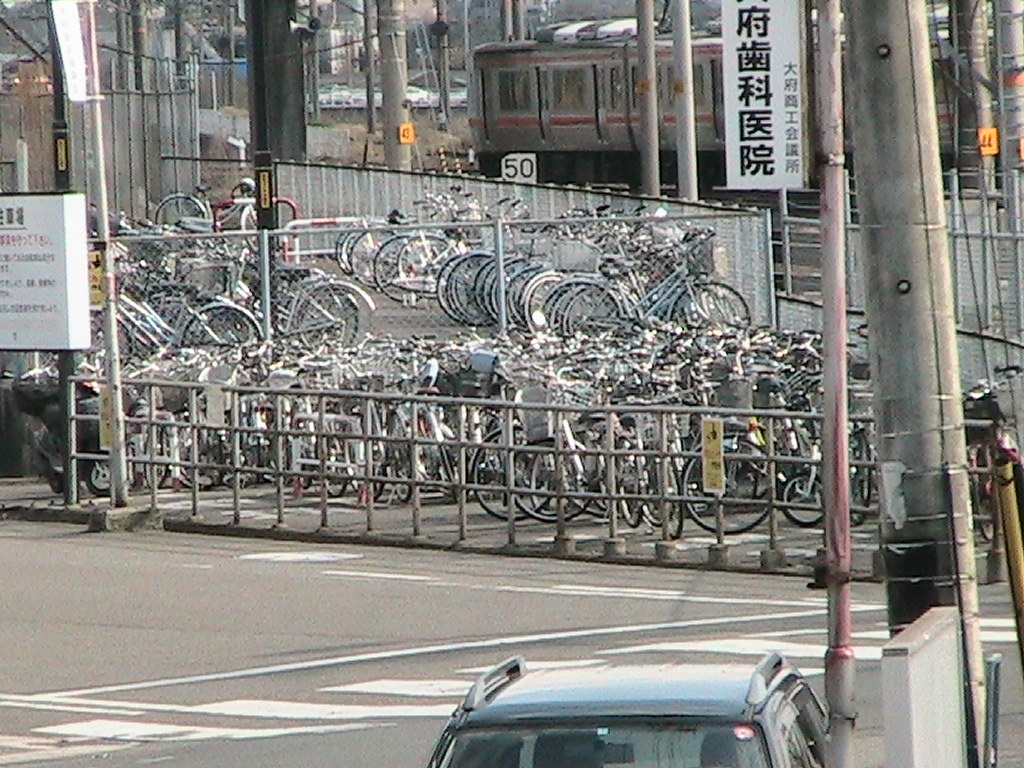In this realistic outdoor photograph, which captures a sunny and bright day, the foreground features a street with part of a parked car visible at the bottom right. Dominating the midground are various fences, including chain-link and shorter metal ones, surrounding a concrete lot filled with an estimated 100 to 200 bicycles in an array of colors like blue, white, and red. The bicycles are densely packed, their black wheels touching. A scratched red metal pole stands tall on the right foreground, supporting a white sign with Asian characters. In the background, there’s a silver train marked with red stripes and a white sign displaying "50" in black font. The scene hints at an Asian country, evident from the signage language and extensive steel fencing that seems to secure the area, possibly to keep people off the railway tracks.